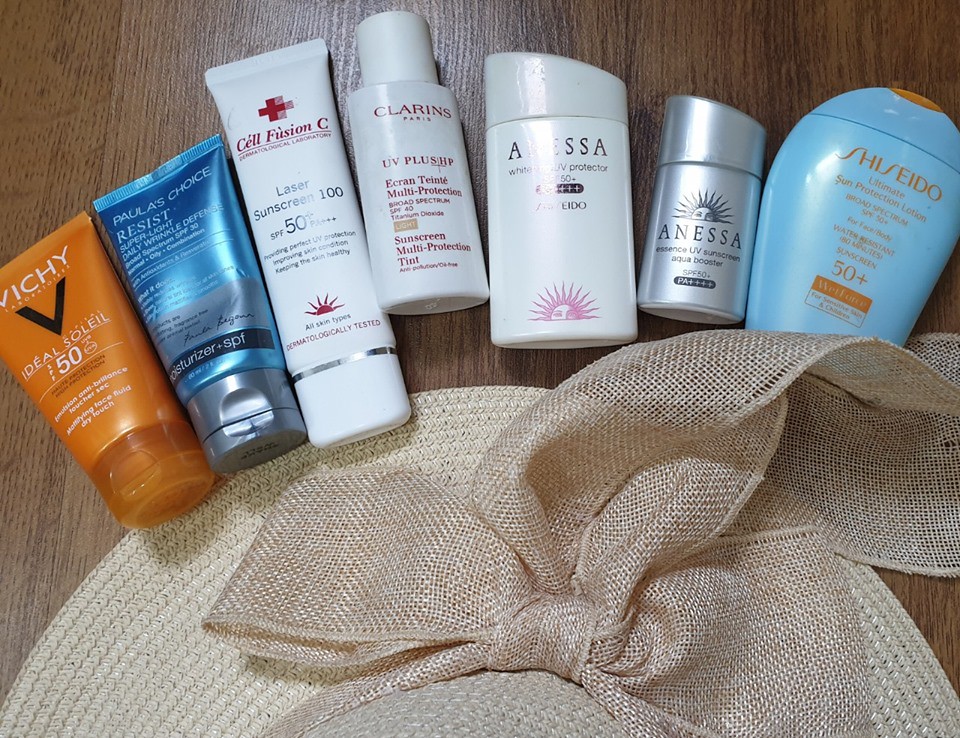In this meticulously arranged photo, a curated selection of seven premium body care products is displayed alongside a charming straw hat adorned with a bow. Starting from the left, the collection begins with a vibrant orange container housing a 50 SPF cream. Next, a sleek bottle of Paula's Choice Resist, an SPF moisturizer, stands prominently. The third item is a sophisticated tube of Cell Fusion C, also boasting a 50 SPF. Midway through the lineup is Clarins' tinted sunscreen with SPF 40, exuding elegance and functional beauty. Following this, a compact and versatile SPF 50 sunscreen by Shiseido makes an appearance. The penultimate product is Anessa's innovative SPF 50 sunscreen, enhanced with an aqua booster for superior protection. Concluding the ensemble is another Shiseido creation, a 50+ SPF sun protectant lotion, offering top-tier sun defense. This entire collection rests gracefully on the floor, perfectly complemented by the stylish straw hat, adding a touch of summery flair to the scene.